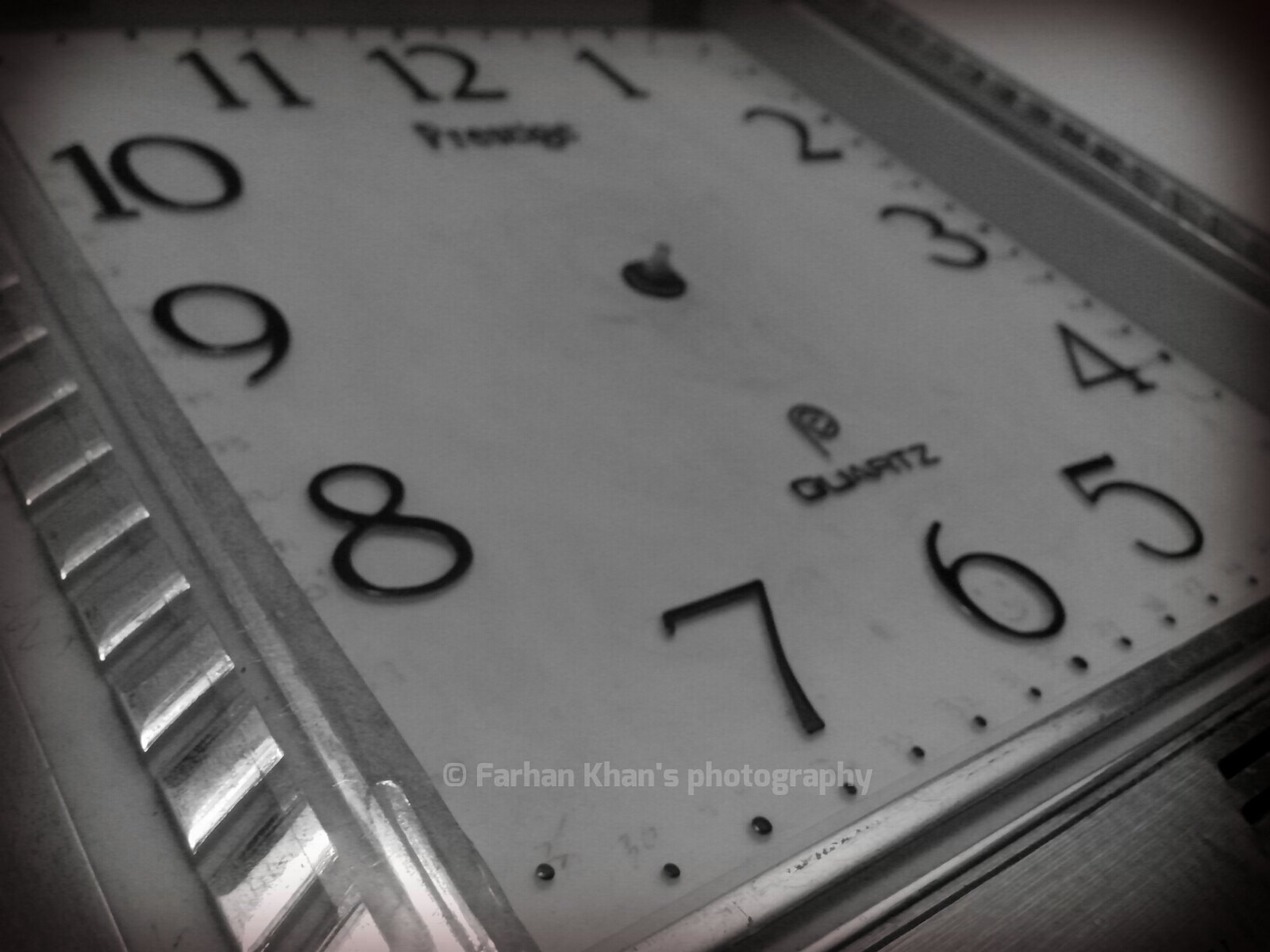This close-up photograph features a watch face with a minimalist, square design. The watch face is detailed with bold, black Arabic numerals, clearly marked from 1 to 12. Notably, the watch lacks hour and minute hands, giving it a modern, sleek appearance. Positioned above the numerals 7, 6, and 5, the brand name "QUARTZ" is prominently displayed in uppercase black letters, adding a distinctive touch. The watch casing is metallic silver, adorned with meticulously patterned square engravings that enhance its texture and visual appeal. In the background, a subtle gray backdrop complements the watch, and at the bottom of the image, a glimpse of the watch strap is visible, seemingly made from a gray fabric, adding to the sophisticated aesthetic of the piece.